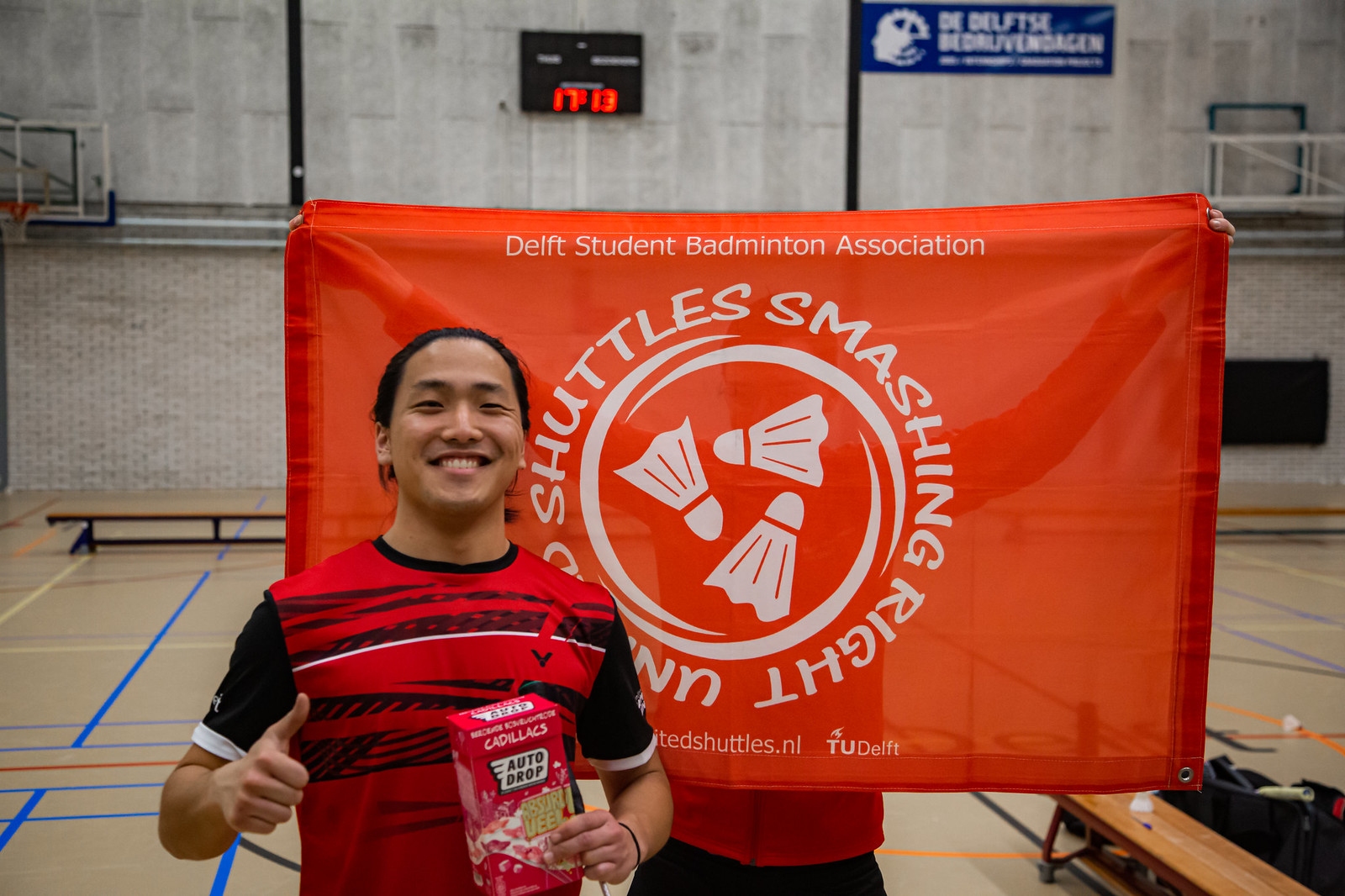In this image, we see a vibrant orange banner with white text at the top reading "Delft Student Badminton Association." The banner features a circular logo in the center with three white shuttlecocks and partially obscured text that appears to say "Shuttle Smashing Right" or similar. The banner is held by someone behind it, whose silhouette and hands are faintly visible through the semi-transparent material.

Standing in front of the banner is an Asian male with caramel-colored skin and black hair pulled back into a ponytail. He is smiling broadly, showcasing his white teeth. The man is dressed in a red jersey with black sleeves and black and white stripes. He holds a red box labeled "Auto Drop" in one hand and gives a thumbs-up with the other, adding to his cheerful demeanor.